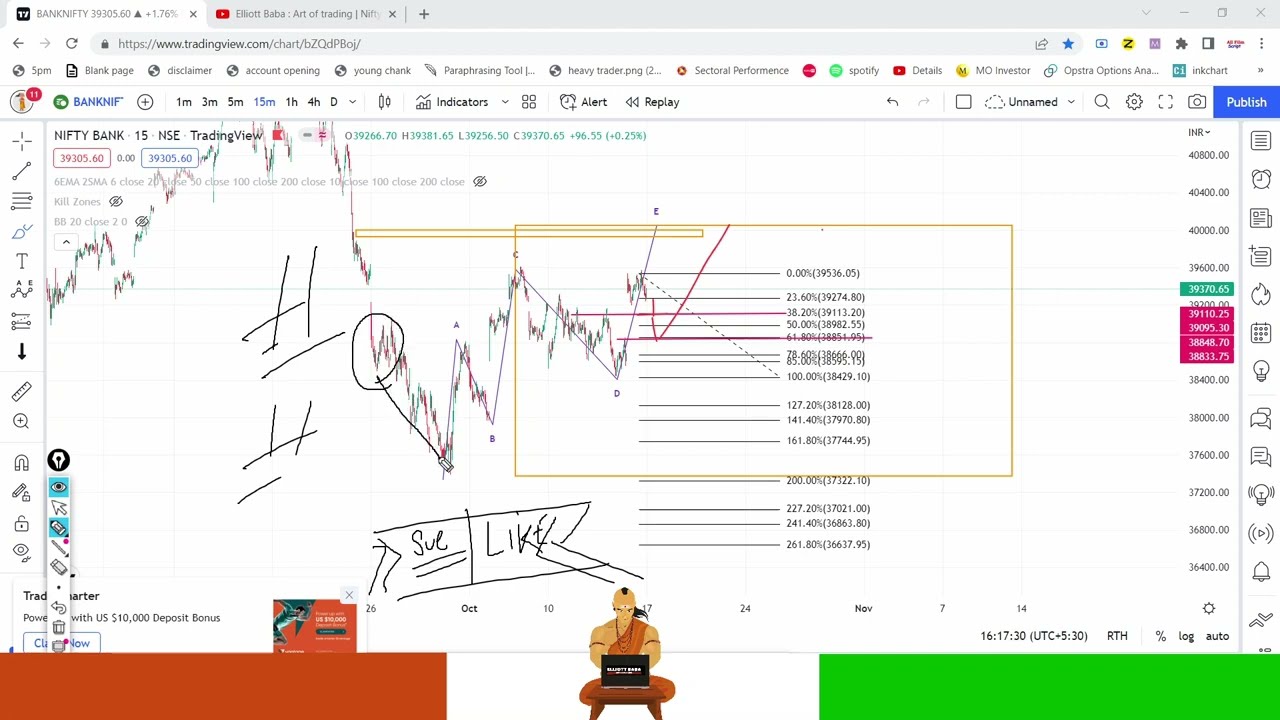This image is a detailed screenshot of a computer screen, primarily displaying a Google Chrome browser open to the "TradingView" website, specifically featuring the "nifty bank" chart from NSE. The title in the upper left reads "BANKNIF." The screen is busy with numerous elements, including a stock market trading price chart that is partially obscured by a variety of drawn lines and scribbles, as if someone used a drawing tool to annotate or obscure parts of it. 

Along the top, there are two open tabs: one for the bank stock information, detailed as "BANKNIF 3930.56 up by 1.76%," and another tab titled "Elliot Baba Art of Trading Nifty" from YouTube. The tabs are nested among a series of bookmarks, which includes links titled "5 p.m.," "Blank Page," "Disclaimer," "Account Opening," "Young Chang," "Paraphrasing Tool," "Heavy Trader," "Sectoral Performance," "Spotify," "Details," "Mo Investor," and "Astra Options."

Details on the chart include faint numbers along the bottom and right side, which are somewhat out of focus. The lower section of the screen features a distinctive bar: an orange bar on the left, a white bar in the center containing a clipart image of a meditative figure reminiscent of an airbender from "Avatar: The Last Airbender," and a lime green bar on the right. The screen also shows a few icons towards the bottom right, including a clock, a flame, a light bulb, and a bell. Overall, the image captures a cluttered and annotated trading interface.